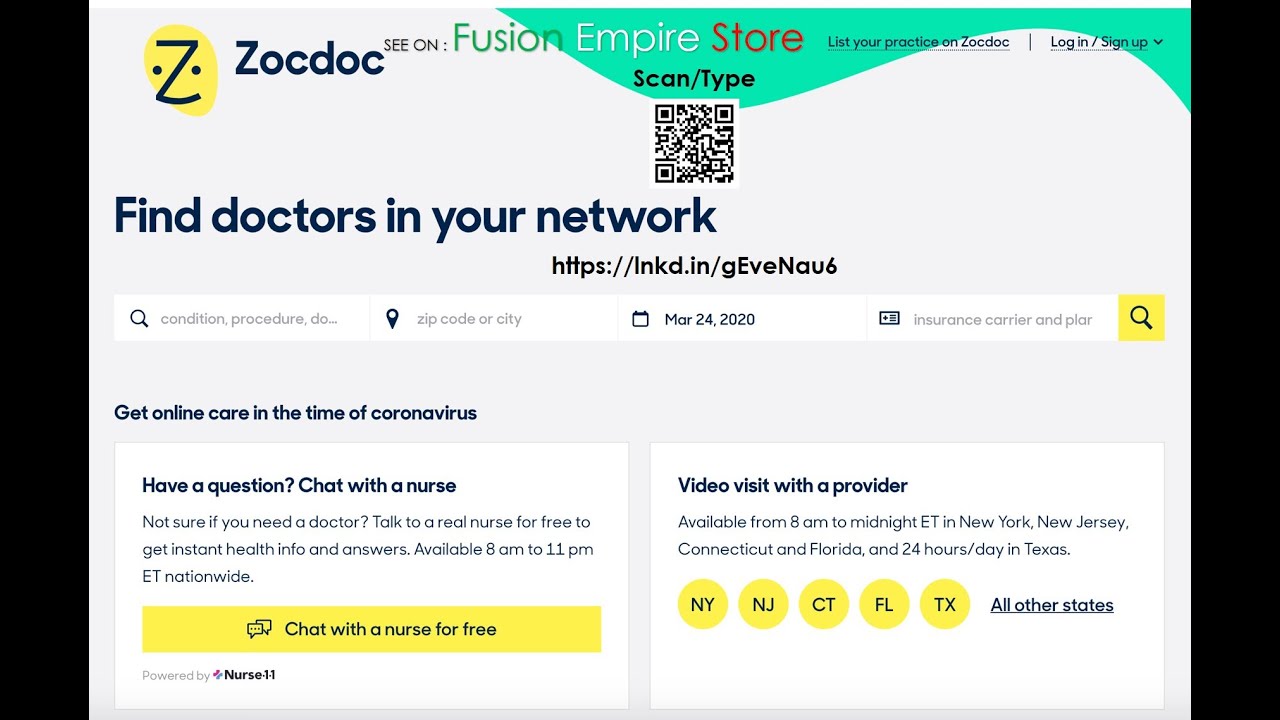This image features a screenshot of the ZocDoc website. In the upper left corner, the ZocDoc logo is prominently displayed - a yellow circle with a dark blue 'Z' in the center, flanked by two dots resembling a smiley face. Adjacent to the logo, text reads "See on Fuze and Empire Store," accompanied by a barcode instructing visitors to "scan/type."

In the upper right corner, there are navigation options including "List Your Practice on ZocDoc" and a dropdown menu for "Log In" and "Sign Up." The main header of the page reads "Find Doctors in Your Network."

Below this header, the image has been altered – an external LinkedIn link (lnkd.in/GevEnAU6) and associated barcode are conspicuously pasted onto the page. This suggests that the screenshot has been used to promote the LinkedIn profile, likely leveraging the ZocDoc platform's credibility for personal advertisement.